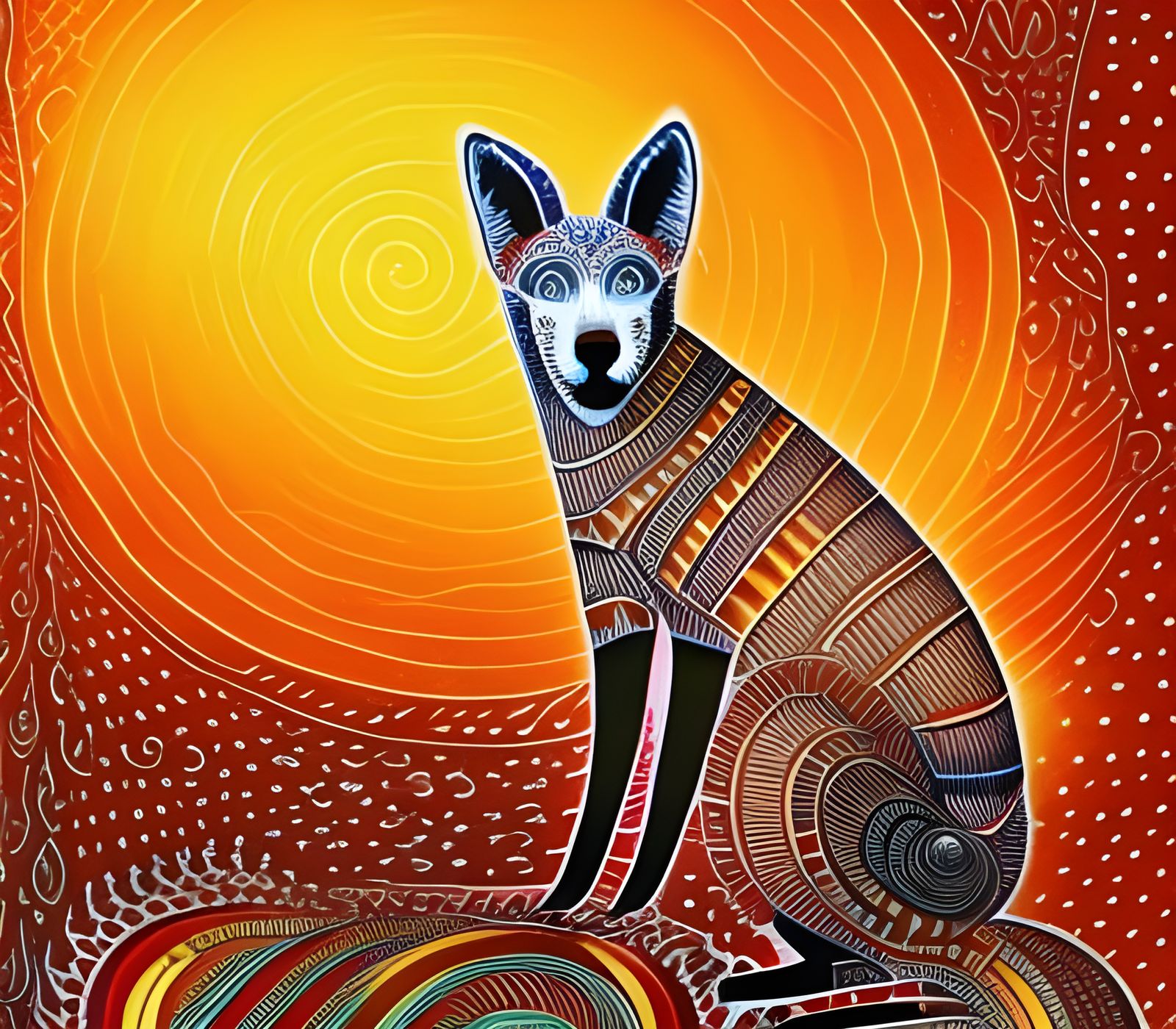This painting features miraculously vivid colors and presents an artistic interpretation of the sun in the background, characterized by a large, swirling spiral of various shades of orange transitioning from a darker hue on the outer edges to a lighter yellow-orange at the center. The sun, which occupies about two-thirds of the image, is surrounded by red patterns including wiggles, squiggles, dots, curls, and white etchings that blend seamlessly with the vibrant backdrop. Overlaid on this radiant sun is the central focus of the piece: a vivid creature resembling a fox, dog, or wolf, portrayed in a distinctive tribal or folk art style. The creature’s body is segmented with intricate lines, patterns, and swirls, incorporating colors like red, orange, black, and blue. Its face, predominantly white with a realistically depicted nose, features strikingly swirled blue eyes giving it a mystical appearance. The creature, with black legs and an almost armadillo-like textured body, faces the viewer with a seemingly pleasant demeanor, against the backdrop of what appears to be an intensely hot and warm desert landscape.